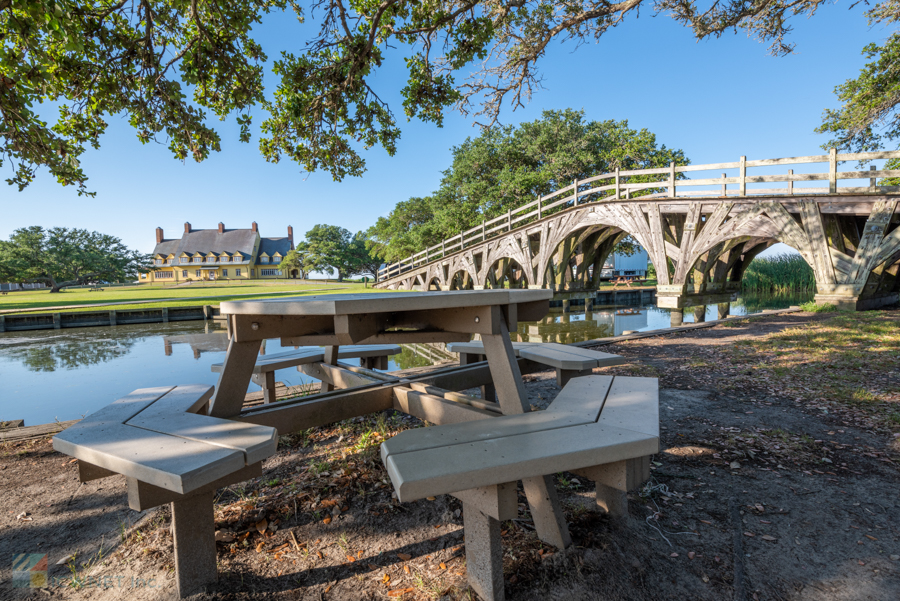This is a detailed photo of an outdoor park taken on a bright spring or summer day. In the foreground, there is a picnic table surrounded by four benches, located underneath a leafy tree beside a canal. The scene is set alongside a manicured river trail. Dominating the middle of the image is an intricately carved wooden bridge that spans the canal, providing a charming passageway to the other side of the park. Beyond the bridge lies an expansive, open green field dotted with mature oak trees and a weeping willow reflected in the canal's waters. This field leads to a two-story, yellow farmhouse or manor with multiple chimneys and numerous windows, capturing the essence of a vast farming estate.